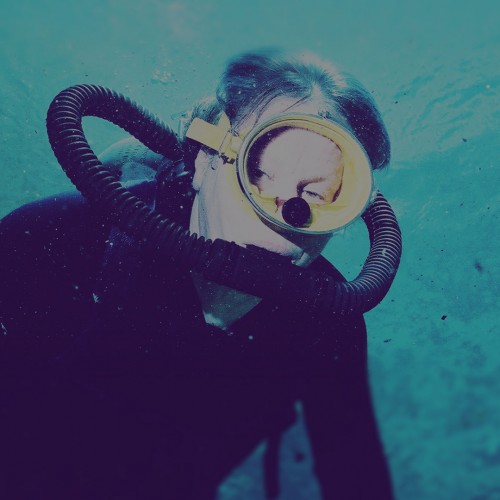The image captures a close-up view of a light-skinned man snorkeling underwater. He is wearing a black diving suit and a yellow face mask with circular goggles. Black tubes extend from his mouthpiece, looping around his back, suggesting the presence of an oxygen tank. The background is a serene blend of blue and green shades, indicating the underwater setting. Despite not being of the highest quality, the image provides ample detail, showing the subject's short brown hair and the sparkling clarity of the water around him. The overall lighting is bright enough to distinctly illuminate the scene.